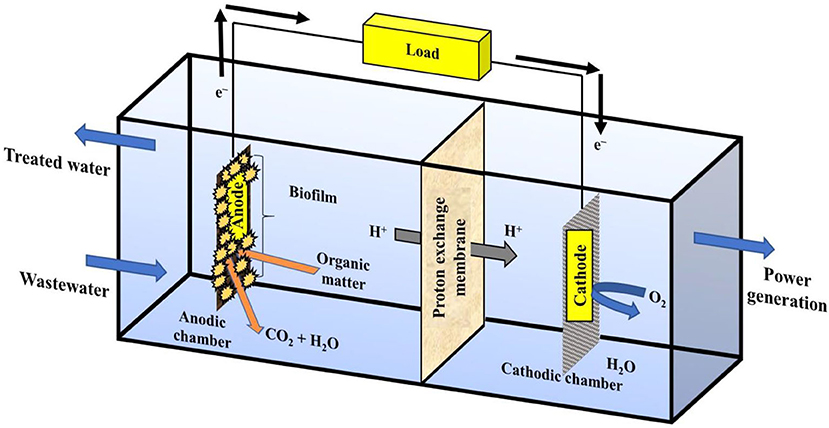The image is a detailed schematic diagram, resembling an instructional chart, illustrating the process of wastewater treatment and power generation. At the top of the diagram, there is a three-dimensional yellow rectangular object labeled "load," with lines extending from it to both sides and then downward into a larger box. This larger box is divided by a "proton exchange membrane," creating two chambers.

On the left side of the membrane is the "anodic chamber," which contains labels such as "biofilm," "organic matter," "anode," along with CO2 + H2O. Arrows within this chamber indicate the flow of wastewater entering the system and the treated water exiting it. The anodic chamber is designed to facilitate the breakdown of organic matter.

On the right side of the membrane is the "cathodic chamber," which includes a "cathode" label. This chamber also shows O2 involvement and an arrow indicating the flow of H2O. An arrow from this chamber signifies power generation, highlighting the dual function of the system in both treating water and generating power.

Overall, this diagram effectively integrates components such as the anodic and cathodic chambers, biofilm, organic matter, and proton exchange membrane, all crucial for the dual processes of water treatment and power generation.